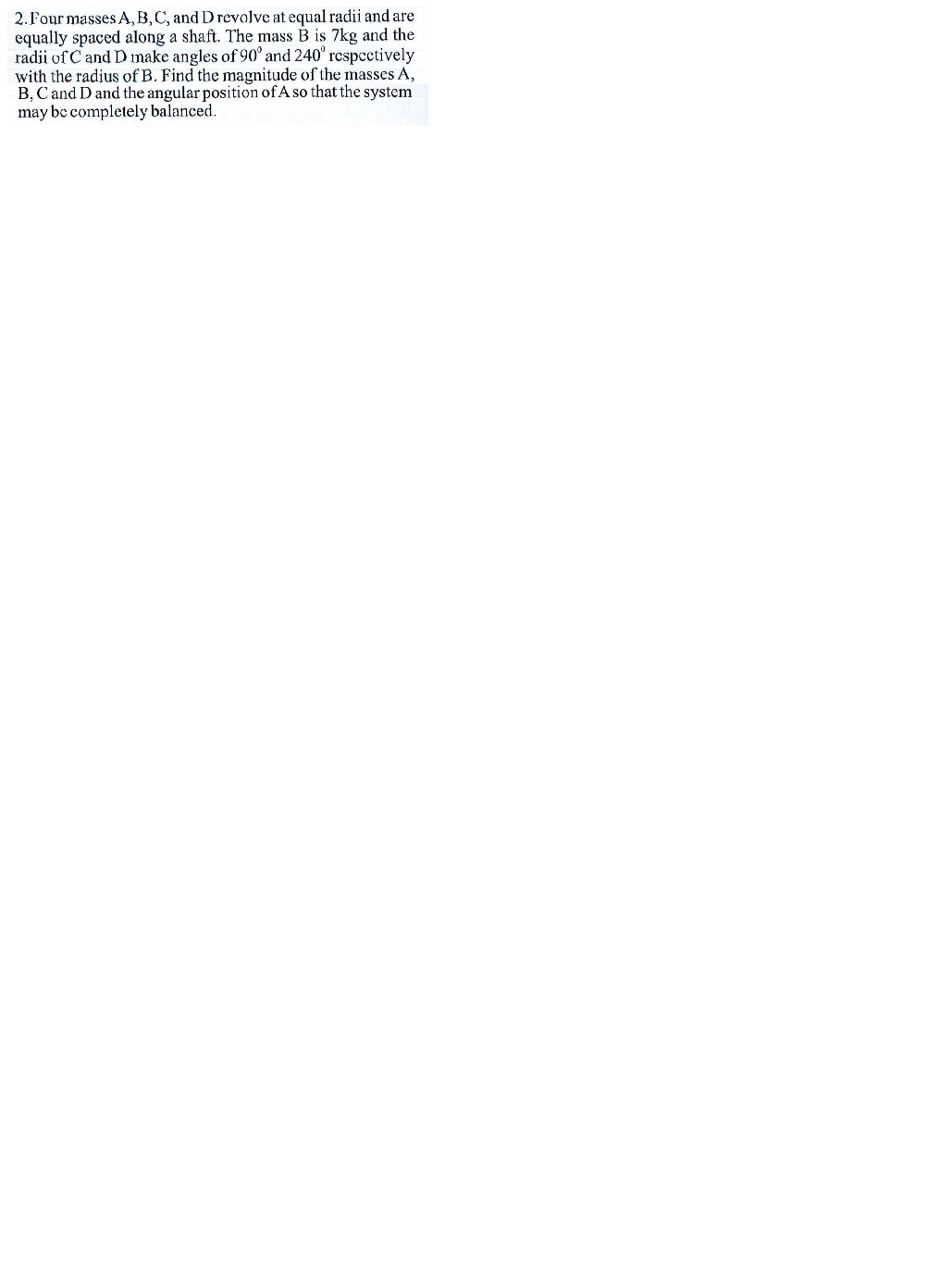This image is a scanned page from what appears to be a textbook on physics or chemistry, potentially aimed at college or school students. The passage, presented in black Times New Roman font, details a problem involving four masses, labeled A, B, C, and D, which are rotating at equal radii and are evenly spaced along a shaft. The text specifies that mass B is 7 kilograms, with radii of C and D forming angles of 90 degrees and 240 degrees respectively with the radius of B. The problem requires finding the masses of A, B, C, and D as well as determining the angular position of A to achieve a completely balanced system. The excerpt seems to be a typical exercise found in educational materials, likely related to topics in physics, chemistry, or mathematics. The background suggests it is copied from a white piece of paper, likely from a textbook or lab manual.